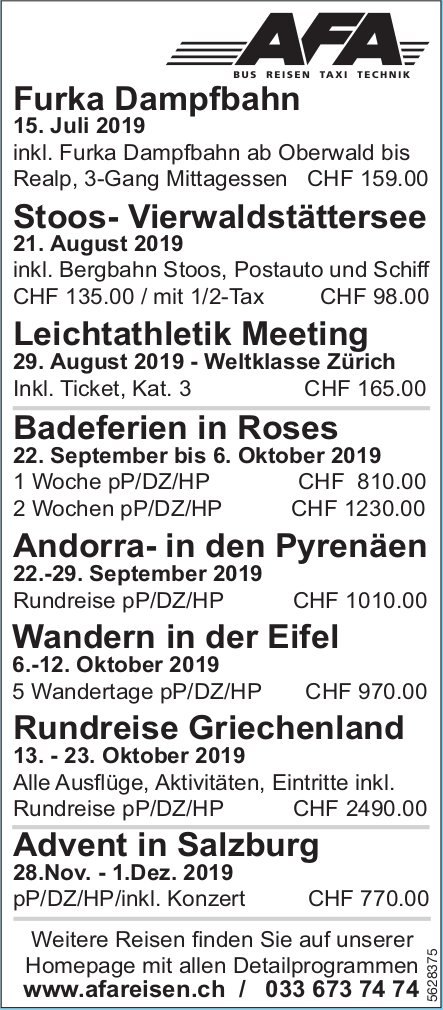The image displays a detailed schedule or menu in a non-English language, possibly German. At the top, there is a logo with the letters "AFA" in bold black font, flanked by four horizontal lines on each side. The schedule lists various events or activities, each associated with a specific date in 2019. The dates range from July to November, starting with "15. Juli 2019" and including notable entries such as "Ferke Dampfungbahn," "Stus Vir Waldstattersee," and "Advent in Salzburg." The thin blue lines divide the text into sections. At the bottom, there's a website URL, "www.afareisen.ch," and potentially a phone number, indicating contact information. The overall appearance suggests an organized itinerary or promotional material for a series of events or trips.